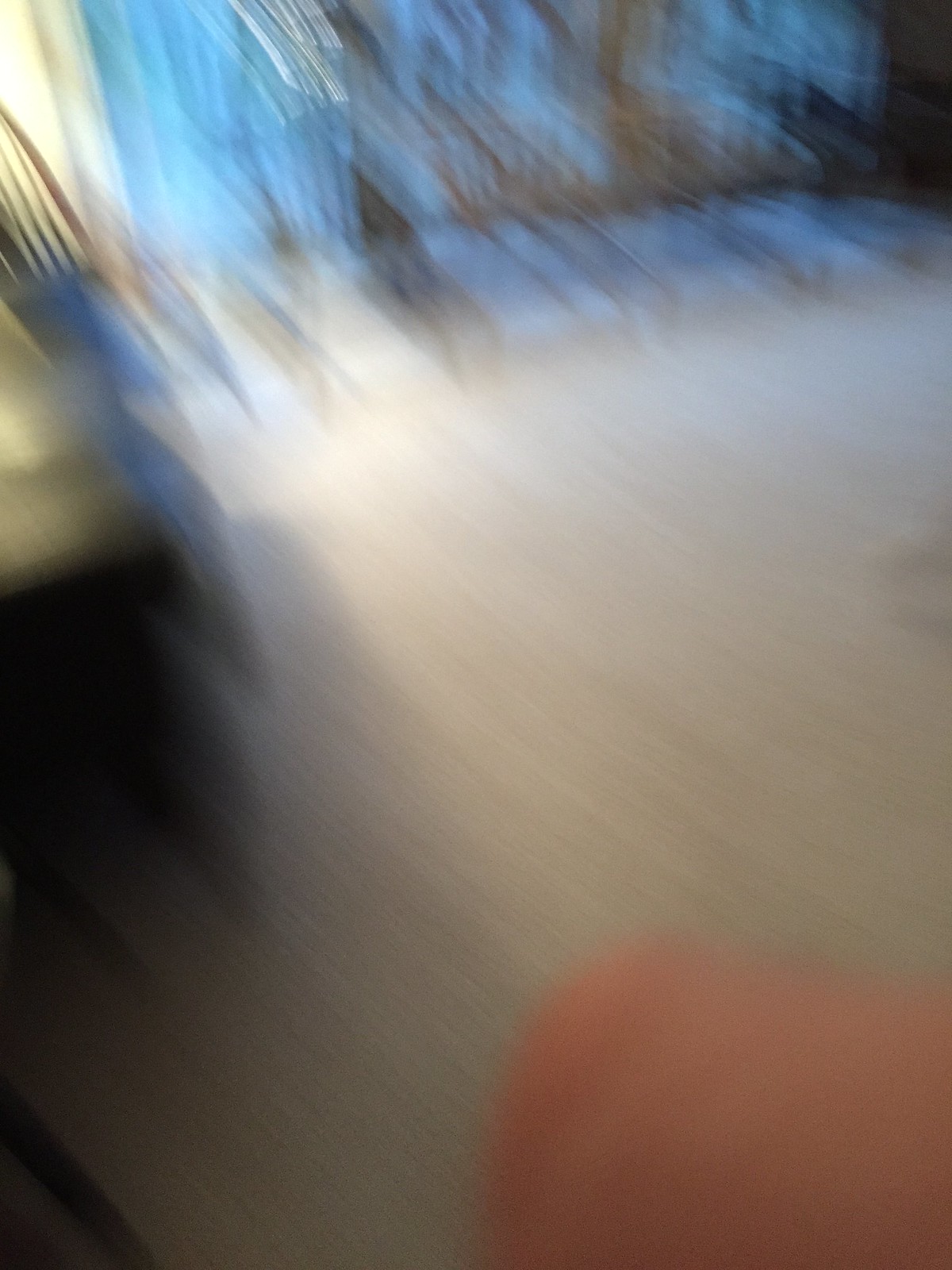This image is an extremely blurry photograph likely taken when the camera was in motion, resulting in an abstract and complex scene. The color palette includes shades of blue, white, brown, gray, and almost black, with some flashes of orange in the bottom right corner. The primary foreground appears to depict part of a living room or a similar indoor setting. In the lower right corner, there's a noticeable skin tone shape resembling a person's knee, potentially that of a Caucasian individual. Adjacent to it, there is a red semicircle and small brown object which might be associated with the floor, hinting that it could be light-colored wood. On the lower left, there's a texture that appears to be a wood grain, possibly indicating the edge of a wooden table transitioning to a darker shaded floor.

The upper portions of the image indicate the blurred outlines of furniture or structural elements, potentially suggesting a staircase or a piece of furniture on the upper left edge. Further above, there's an impression of a wall of windows with natural light filtering through, possibly covered by blue curtains that seem to be fluttering in the wind, adding a dynamic element to the scene. The overall image is intriguing yet indistinct, with reflective surfaces and semi-translucent details making it challenging to definitively interpret the full context of the scene.